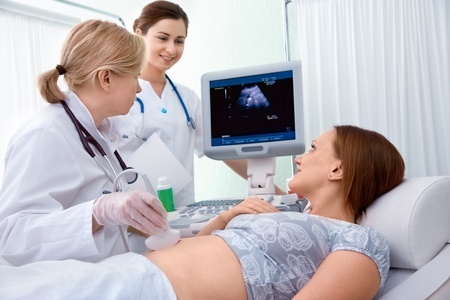A woman with dark brown hair and fair skin is lying on a hospital bed, her head positioned towards the right. She's wearing a mixture of light gray and dark gray tops, partially pulled up, with a hospital gown covering her lower half. Two female doctors are attending to her; a blonde doctor in a ponytail is seated beside the bed, using an ultrasound probe on the woman's stomach, while a brunette doctor stands nearby, observing the ultrasound monitor. The woman on the bed appears to be pregnant and is engaging in conversation with the standing doctor; both are smiling. High-tech medical equipment, including a computer monitor displaying the ultrasound image, is arranged around them, creating a professional and supportive atmosphere.